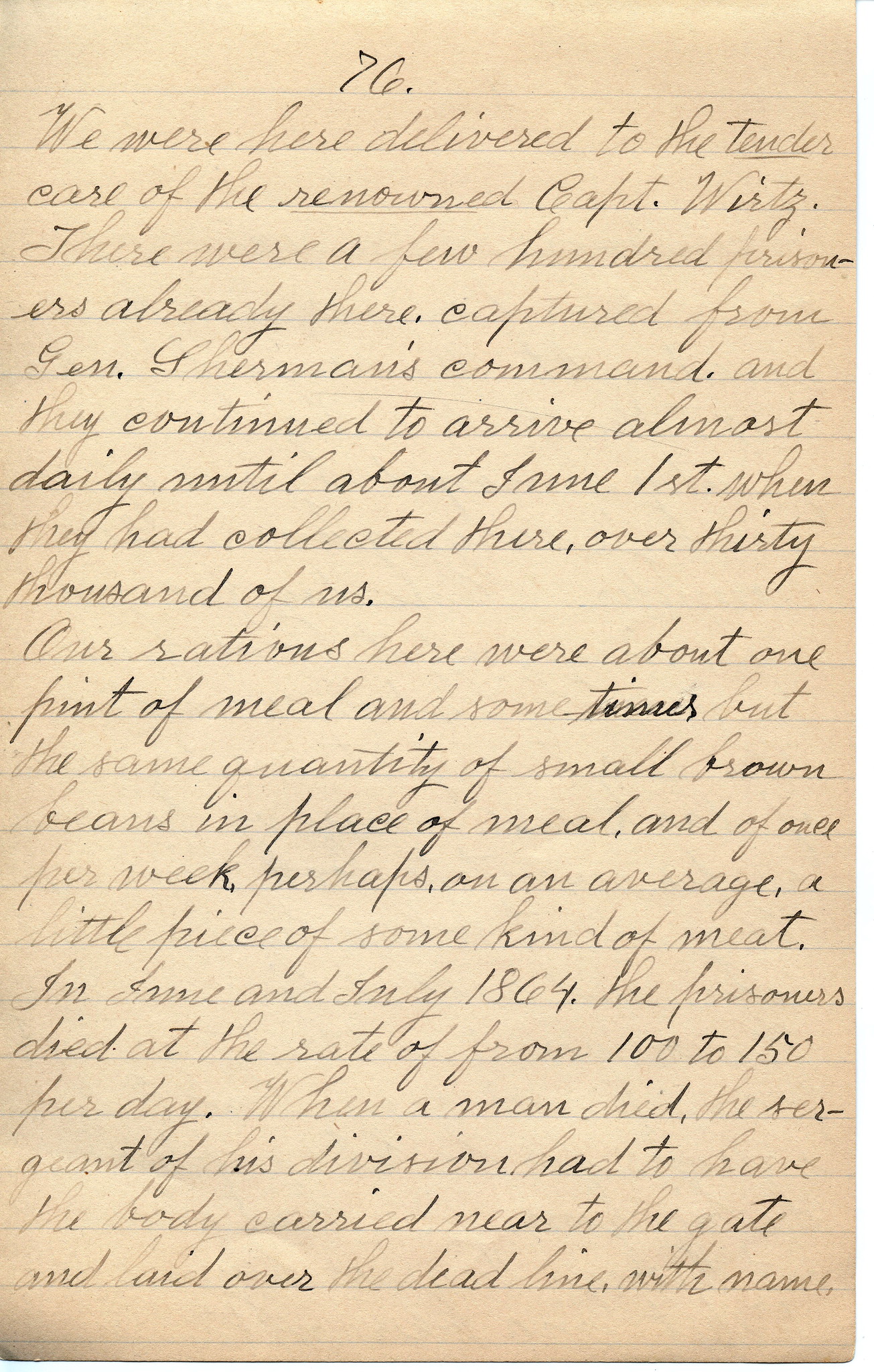This photograph showcases an aged handwritten letter on beige paper, with faded text hinting at its historical nature. The letter features very ornate and surreal cursive handwriting, the kind rarely seen today, written in black ink. The text is slanted and composed of two to three paragraphs, with each word meticulously inscribed, though parts of the letter have become difficult to read over time. The paper itself has thin blue lines, suggesting it came from a notebook, and the top of the letter is marked with the number "76." Key phrases such as "We were here, delivered to the tender care of the renowned Captain Wirtz" and mentions of "prisoners" and "rations" weave a poignant narrative indicative of historical hardships. Despite the challenges in reading the entire text, the delicate and intricate handwriting offers a glimpse into the past, evoking a sense of authenticity and nostalgia.